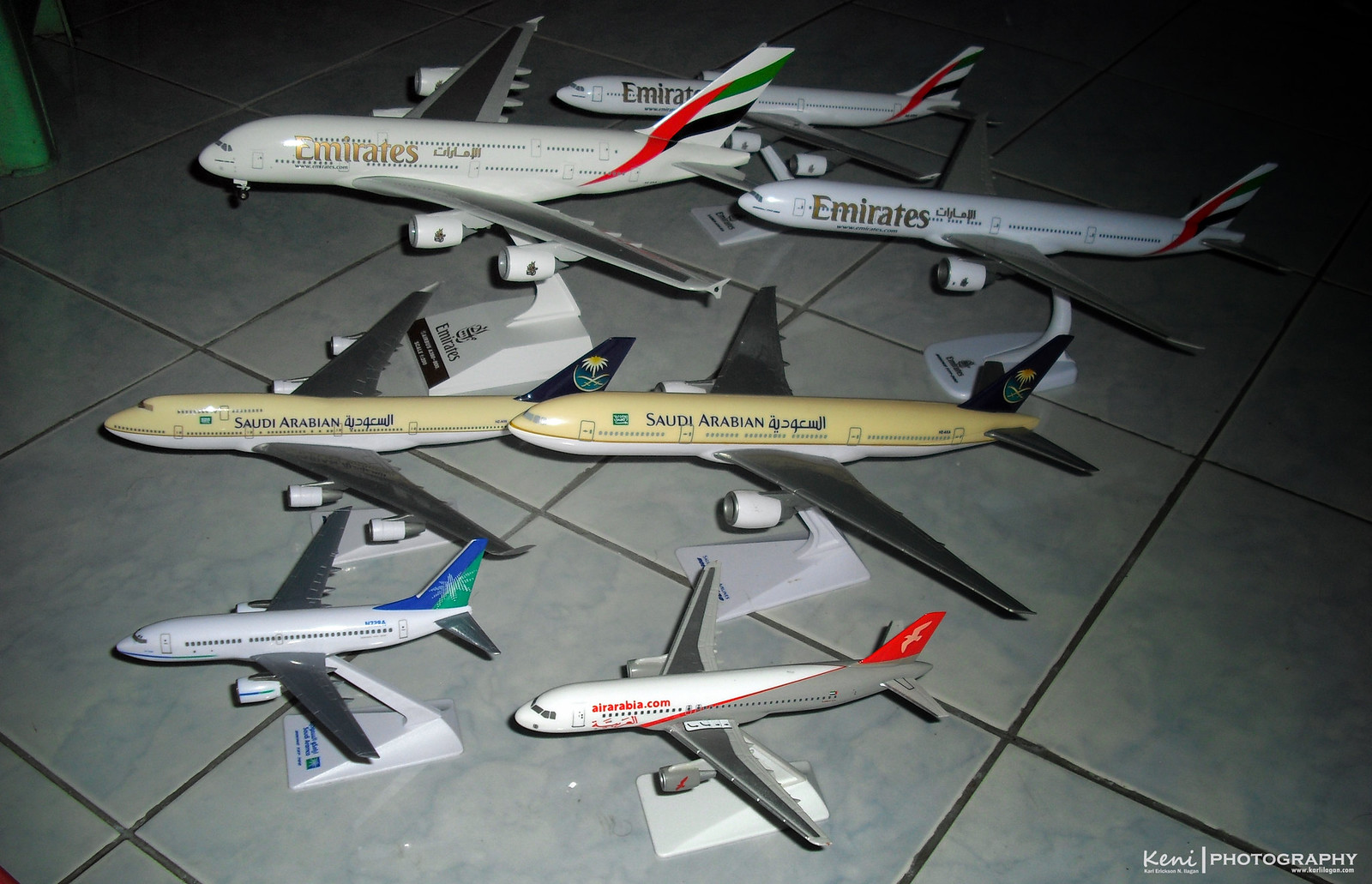This image features a collection of seven small model airplanes meticulously arranged on a mottled gray tiled floor. The tiles have dark grout lines and the photo seems to be taken with a flash, making the center bright while the edges appear darker. Starting from the bottom, the frontmost airplane displays "airarabia.com" in red text, its body a mix of white and gray, with red detailing on the tail. Directly above it, there are two Saudi Arabian airplanes featuring tan tops and white bottoms, positioned side by side. In the middle rows, you will find two pairs of Emirates planes—one Emirates plane on the left and one on the right in each row—with slightly different shades; the left one is a cream color while the right is white, and the topmost single Emirates airplane is also white. Additionally, up in the top left corner of the image, there is a mysterious lime green object, the nature of which is unclear. Each of the airplanes is mounted on a small stand which lifts them slightly off the ground. The photograph is credited to "Kenny Photography," noted in the bottom right-hand corner.